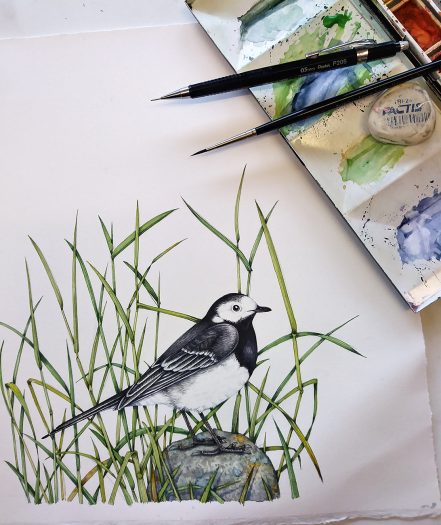This is a detailed image of a watercolor painting on a large, white piece of paper. The focal point of the painting is a medium-sized bird standing on a gray rock surrounded by tall, sparse green grass, which includes various shades of green mixed with some yellow. The bird is intricately detailed with a white belly and a black throat, a short black beak, a white mask around its eyes, and wings that are black with white tips. The feathers on the bird’s wings are particularly well-defined. Additionally, the bird has black legs and a pointed, sharp tail. 

In the upper right corner of the image, there is a dish with individual trays of watercolors, featuring a mix of greens and blues, alongside a mechanical pencil, a fine paintbrush, and a large white eraser. Further into the far right corner, depleted paint palettes can be seen, contributing to the artistic atmosphere of the scene. The bird and the rock are positioned at the bottom center of the paper, creating a balanced and lifelike composition.